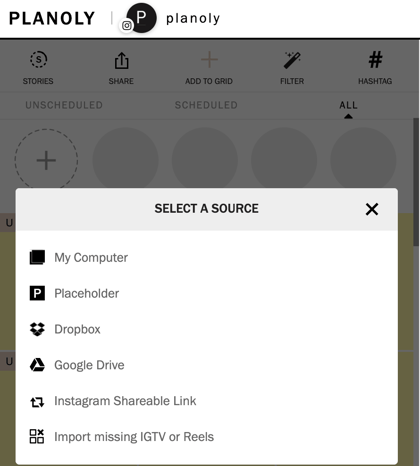In the foreground of the image, we see a Planuli. Behind the Planuli, a row of stores lines the background. The interface includes various options such as "share," "add to," "grid," "filter," and "hash tag," along with a series of choices like "unscheduled," "scheduled," "all," and "select a source." Available sources are listed as "my computer," "Dropbox," "Google Drive," and "Instagram shareable link." Additional options include "import missing IGTV or reels." The overall color scheme of the interface is predominantly white and black. Notably, there are no reticles present on the page.